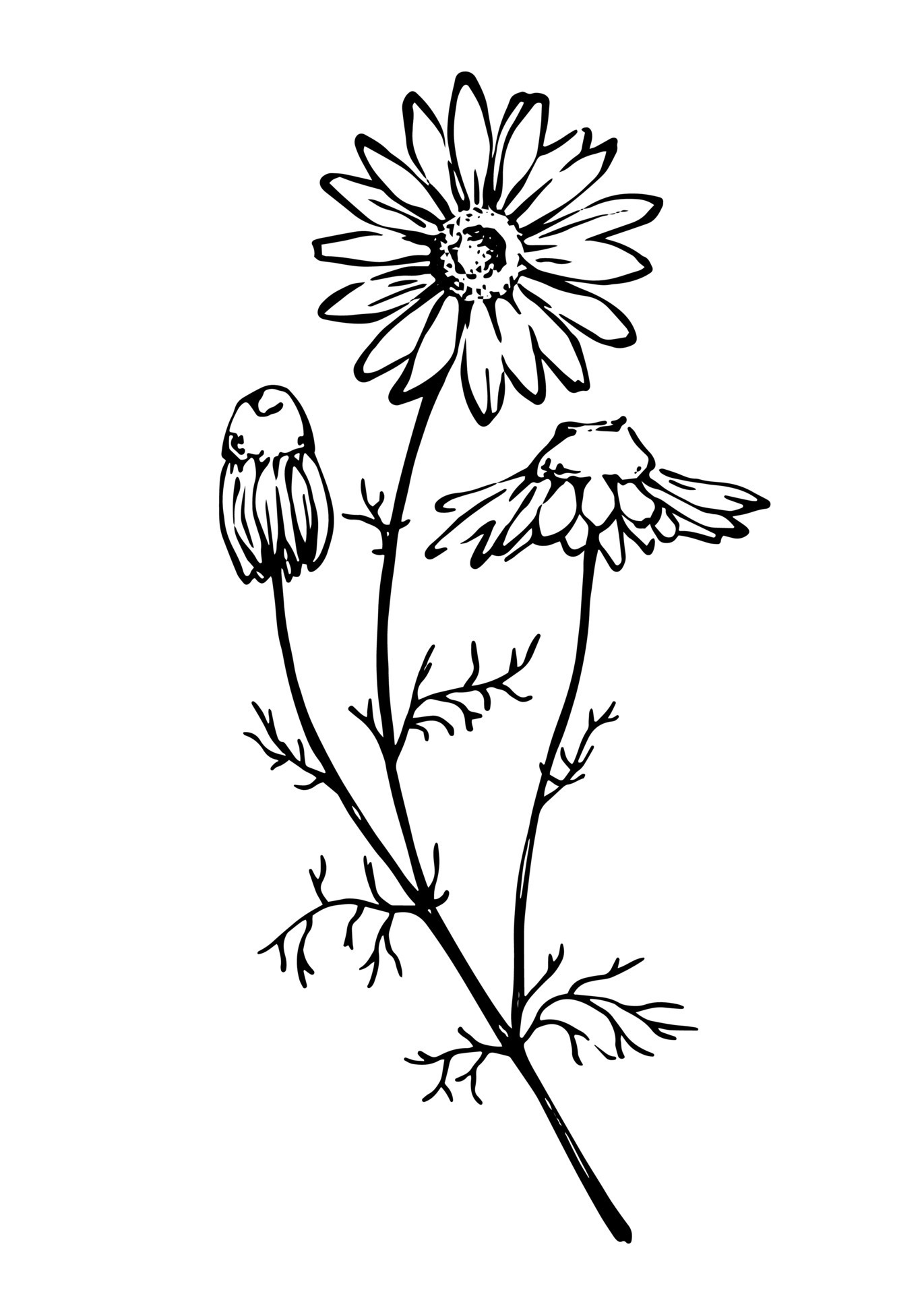This detailed black-and-white drawing features a simple white background highlighting the stark black ink used for the illustration. The image showcases a single stem with three distinct flowers in various stages of bloom. The middle flower, fully blossomed, displays numerous intricately drawn petals. To the left, a flower remains in its bud stage, yet to open. The right flower is partially sprouted with visible petals. Several smaller branches or twigs extend out from the main stem, adding complexity to the drawing. The clean, monochromatic nature of the illustration makes it an ideal candidate for colorization.